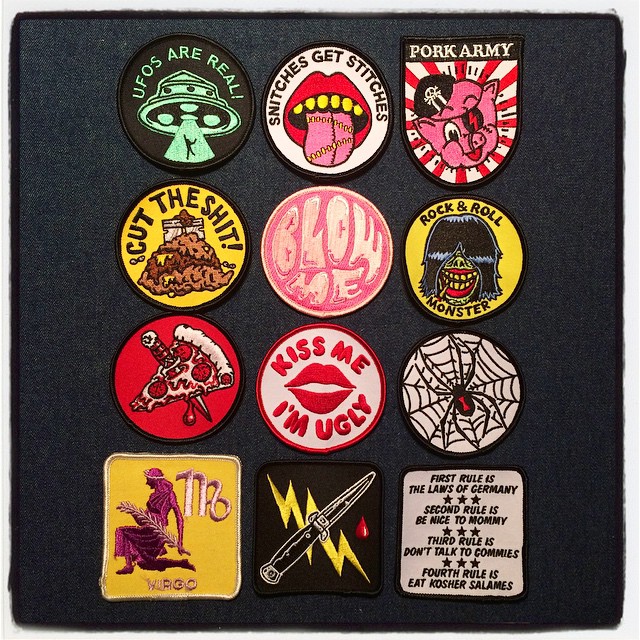The image shows twelve diverse and novelty embroidered patches arranged on a black felt background. Starting from the top left, the first patch features a green UFO beaming up a person with the text "UFOs are real." The second patch displays an open mouth with stitches on the tongue, accompanied by the phrase "Snitches get stitches." The third patch reads "Pork Army" and depicts a pig wearing an eyepatch and pirate hat. The fourth patch shows a razor blade cutting through a piece of poop with the phrase "Cut the shit." Next, a patch reads "Blow me," and the one beside it says "Rock and roll monster," illustrated with a figure with dark hair, big teeth, red lips, and possibly a cigarette. There's also a patch with a pizza impaled by a dagger. Another patch with a white background and bold red stitching says "Kiss me, I'm ugly," featuring large red lips. Another notable patch displays a spider on a spider web. One patch has the letter "M" on it. Another shows a switchblade alongside a lightning bolt. The final patch lists humorous rules: "First rule is the law of Germany. Second rule is be nice to mommy. Third rule is don't talk to commies. Fourth rule is eat kosher salamis."